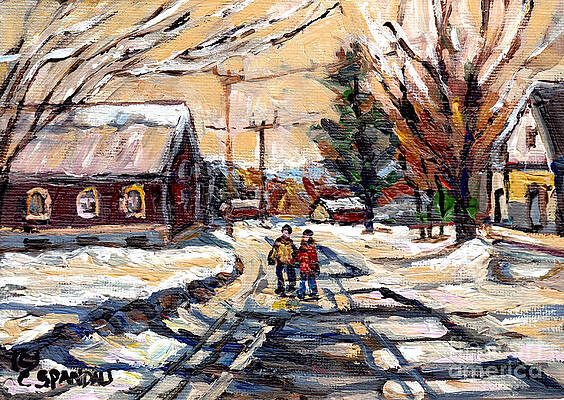This is an oil painting on canvas by an artist named C. Spandau, as indicated by the signature in the lower left corner. The painting portrays a vibrant yet somewhat muted winter scene in a small town. It features two figures, possibly children or a couple, dressed in a red coat and yellow coat with winter hats, walking down a snow-covered street. The expressive brush strokes and abstract style allow for a range of colors, making the scene both simple and richly textured. 

On the left side of the painting, there is a small country church with stained glass windows, flanked by telephone poles. In the foreground on the right, a house stands beside a bare deciduous tree and a pine tree. Further up the street, additional trees and houses are visible, contributing to the charming, serene atmosphere of the town. Snow blankets the entire scene, with tracks visible on the road, leading the eye toward the rolling hills in the background. The sky is painted in a goldish hue, contrasting with the dark reds and white snow, creating a picturesque New England-like winter setting.